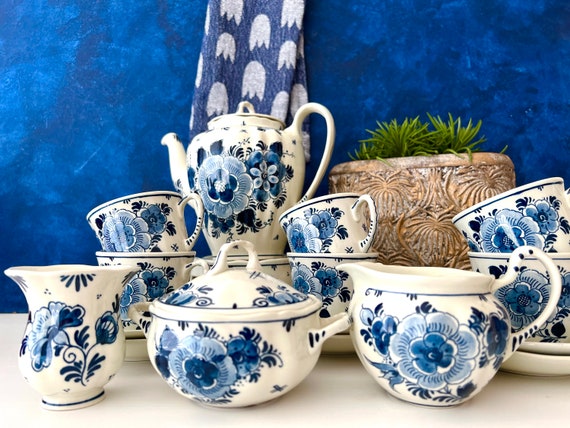This highly detailed image captures an exquisite black ceramic or porcelain tea service adorned with intricate blue floral patterns. The set comprises a teapot, creamer, sugar bowl, and six matching teacups with saucers meticulously arranged on a cream-colored surface. A closer examination reveals a flower pot behind the tea service, featuring a tan base decorated with designs resembling palm fronds and housing a small green plant. The background showcases a navy blue wall, ornamented with what appears to be a towel patterned with light blue and white tulips, which add an elegant touch to the setting. This picturesque arrangement, reminiscent of a spread in Better Homes and Gardens magazine, epitomizes refined elegance and attention to detail.